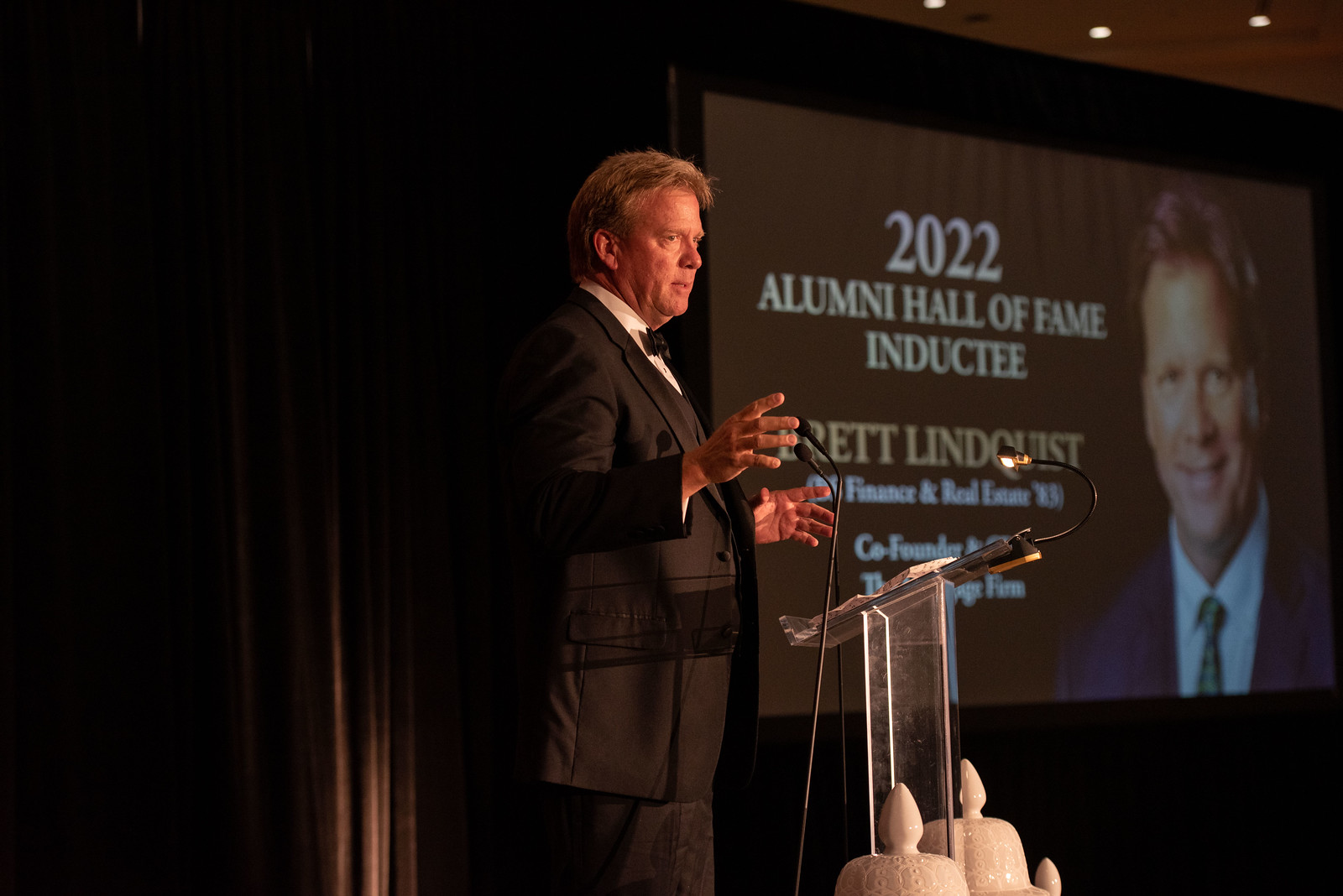The image is a detailed color photograph in landscape orientation, taken indoors in a banquet hall. At the center of the image is a man with a lighter skin complexion, dressed in a formal black tuxedo with a white undershirt and a black bow tie. He stands behind a clear, transparent podium with his hands outstretched, appearing to address an audience. Positioned directly in front of a microphone, he is turned slightly sideways, facing the right side of the image.

In the background on the right side of the image is a projector screen. The screen displays a slide with a photograph of the same man pictured at the podium, alongside text that reads, "2022 Alumni Hall of Fame inductee Brett Lindquist." Additional text mentions his roles in finance and real estate, and he is noted as a co-founder, although this part is cut off. The room appears bright due to ample lighting, emphasizing the black, brown, gray, tan, blue, green, and white colors evident in the composition. Partially visible on the floor in front of the man are two ceramic vases. The photograph emulates a style of representational realism, providing a clear and well-lit depiction of the formal setting.